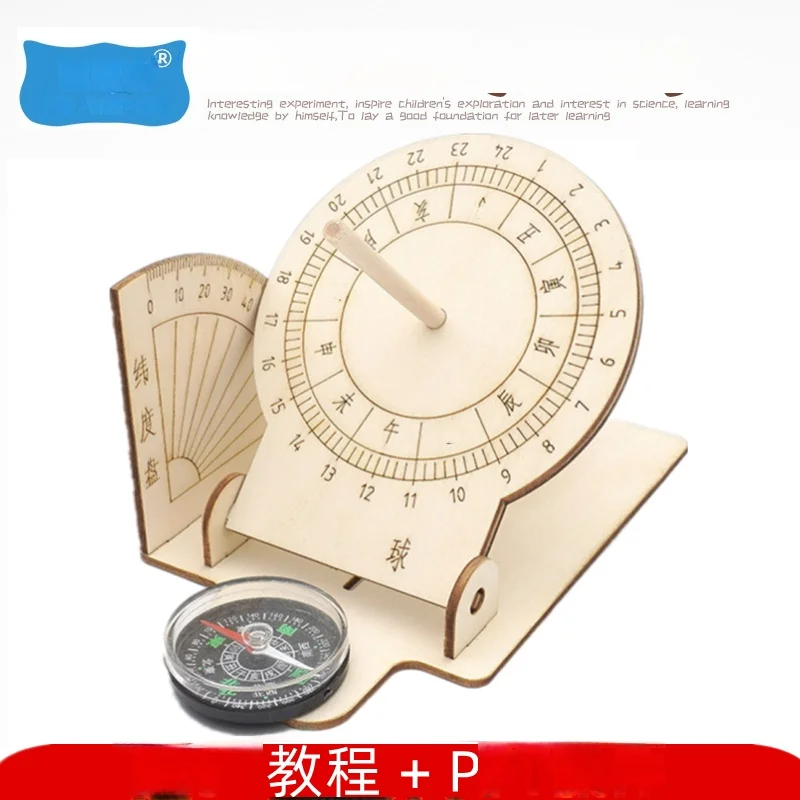The image is a square, color photograph depicting a wooden contraption, resembling a sundial, featuring a plastic compass and a detailed dial. The dial is inscribed with both Asian characters, possibly Chinese or Japanese, and English numbers, suggesting its multinational origin and educational purpose. Notably, the compass is orientated towards north, and the entire setup appears designed to engage children in scientific exploration by teaching them how to use celestial objects for time-telling, aimed at laying a foundational understanding of the subject. At the top of the image, text reads, "Interesting experiment. Inspired children's exploration and interest in science. Learning knowledge by himself to lay a good foundation for later learning." The bottom section of the image features a caption with Asian characters, a plus sign, and a capital "P" on a red background. An obscured blue blob in the top left corner likely covers a logo, reinforcing the idea of an advertisement or product pamphlet aimed at educational enhancement.